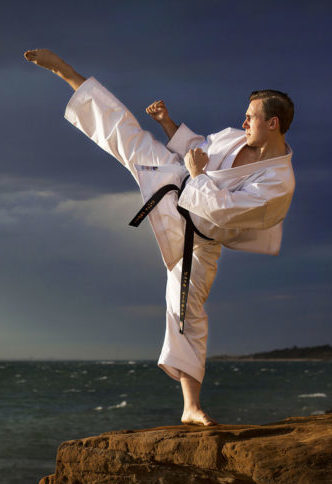In this captivating photograph taken in a vibrant outdoor setting, a man with short dark hair is captured mid-action, executing a high roundhouse kick while balanced on the edge of a rugged, brown rocky cliff. He is dressed in a traditional white karate gi, complete with a black belt, and his fists are clenched, elbows bent towards his target. The man's profile is sharp against a stunning backdrop where the expansive blue ocean meets a sky dotted with white clouds, all illuminated by natural sunlight. The image is presented in portrait orientation, emphasizing the striking contrast between the man's dynamic pose and the serene, yet powerful, natural elements that surround him.